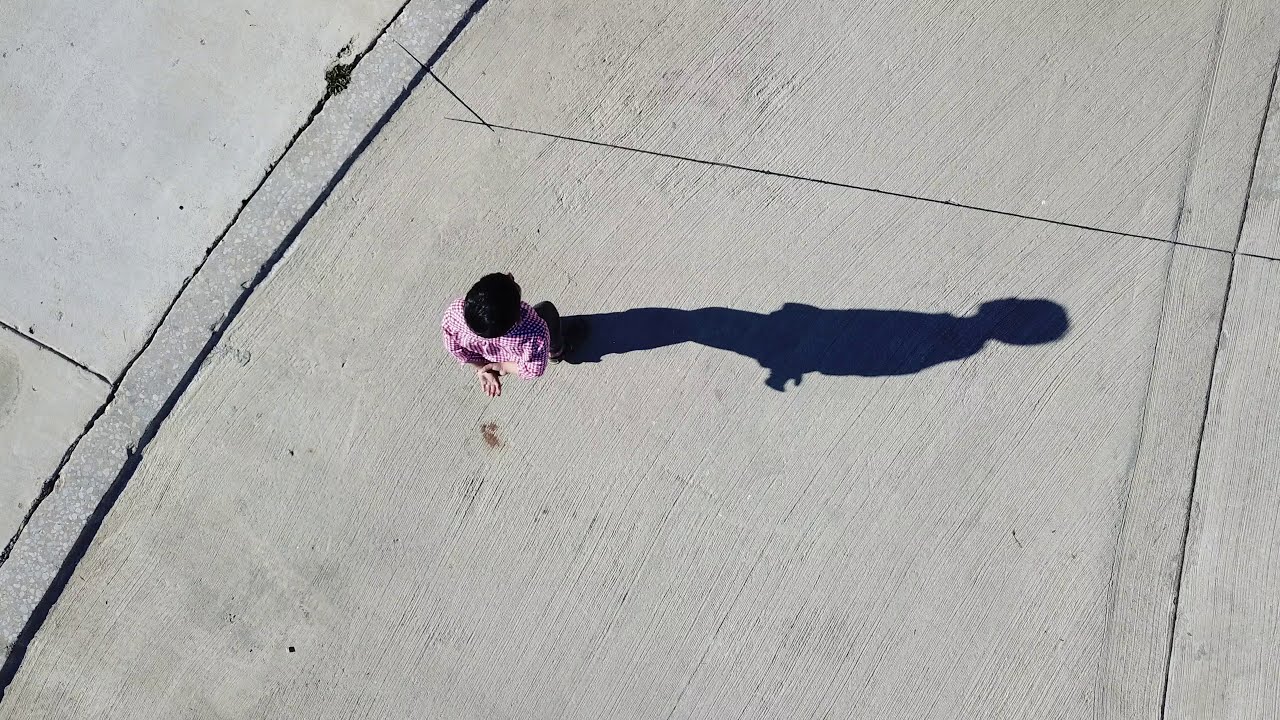This is a top-down, color photograph taken by a drone, showcasing a young man with dark hair standing slightly left of center on a concrete paved pathway, possibly part of a cul-de-sac or a driveway. The man, the main subject of the image, is wearing a red and white plaid shirt and dark pants. He stands with his hands behind his back, his right hand holding his left wrist. The concrete surface around him is textured with visible brush strokes, suggesting it was treated for better traction. His shadow extends to his right, implying the sun is situated to his left. The photograph is in a landscape orientation and captures the overall scene with great realism.